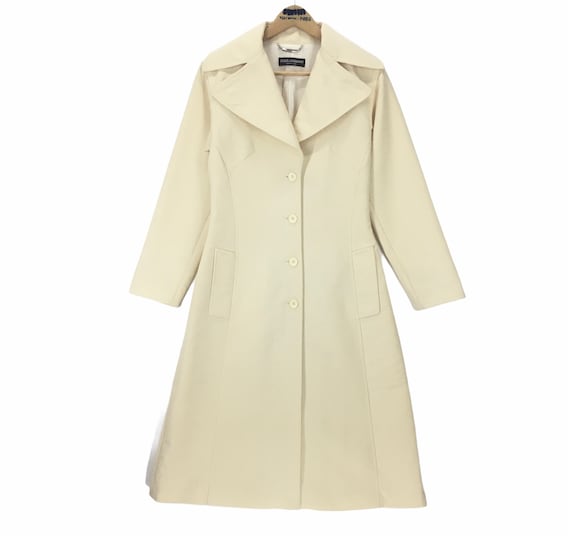The image features a women's trench coat dress in a creamy, vanilla color, giving it a sophisticated yet vintage appearance. The coat is neatly hung on a wooden hanger, which has some small, unreadable text at the top. It showcases a large collar and narrow shoulders, indicative of a feminine style, with sleeves that seem a bit short. The coat is buttoned down the front, with four buttons situated around the torso, leading to a skirt portion that extends further down. There are two flap pockets enhancing its practicality. The backdrop is a simple white, accentuating the coat's subtle yellowish hue against it. The overall image conveys a minimalistic yet elegant presentation, reminiscent of a flight attendant's attire, and suggests detailed craftsmanship.